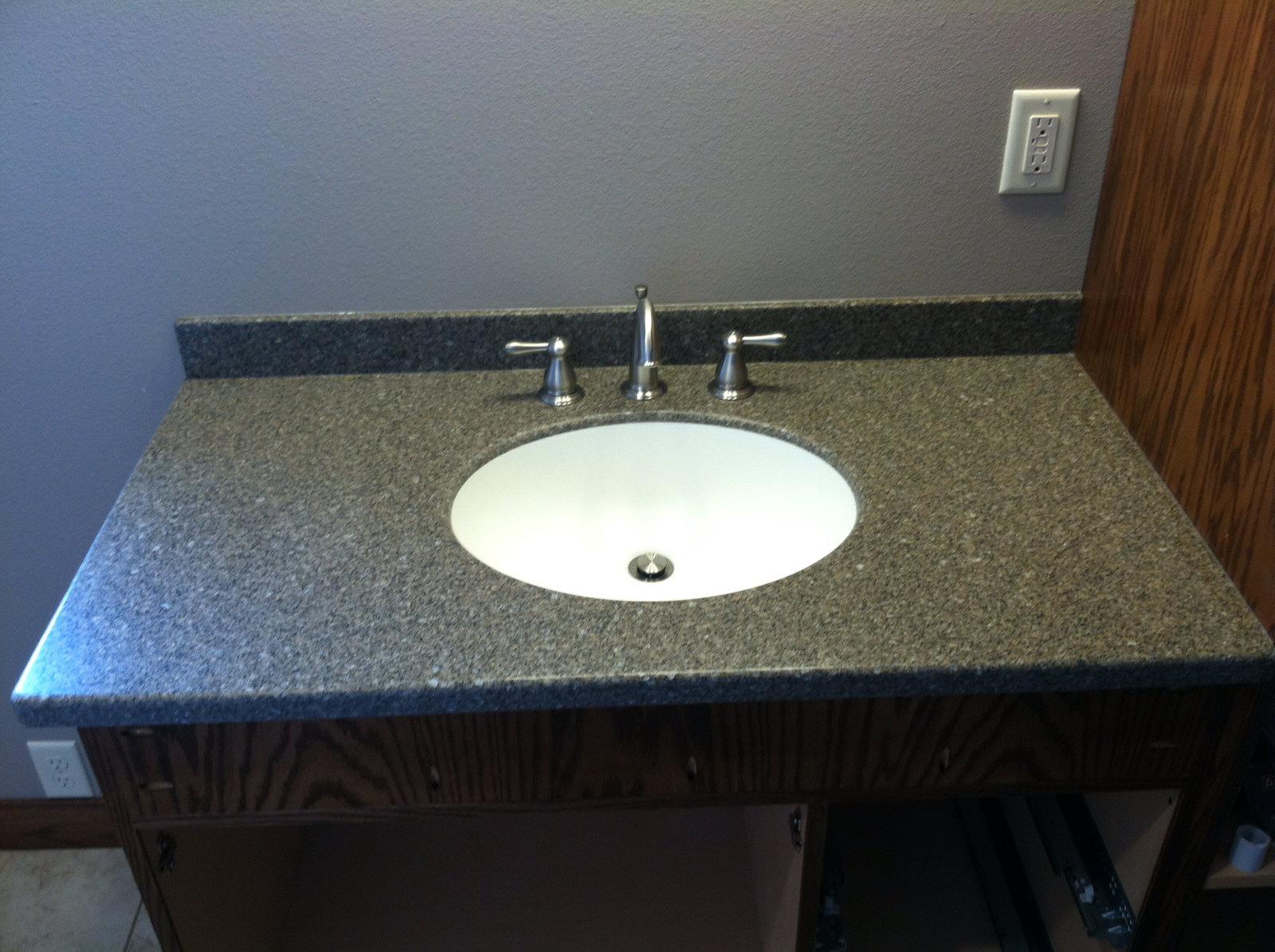This detailed photograph showcases a bathroom countertop with notable elements and distinct finishes. The countertop itself is made of dark gray granite featuring lighter gray and white specks, delivering a sophisticated contrast. The cabinetry below the countertop lacks doors, exposing the interiors and revealing the dark brown wood with pronounced darker grains. On the right side of the image, a wall made of lighter brown cherry wood adds warmth to the space. The wall behind the countertop is painted a shade of gray that, due to the lighting, appears to have a bluish tint. To the left, a white electrical outlet with two sockets is positioned at the junction of the wall and cherry wood segment, and another socket is located at the baseboard. Centrally positioned on the countertop is an elegant white oval sink, equipped with a silver drain. The sink is flanked by a silver faucet and two silver handles, which are oriented outward, enhancing the symmetrical design and modern aesthetic of the bathroom.